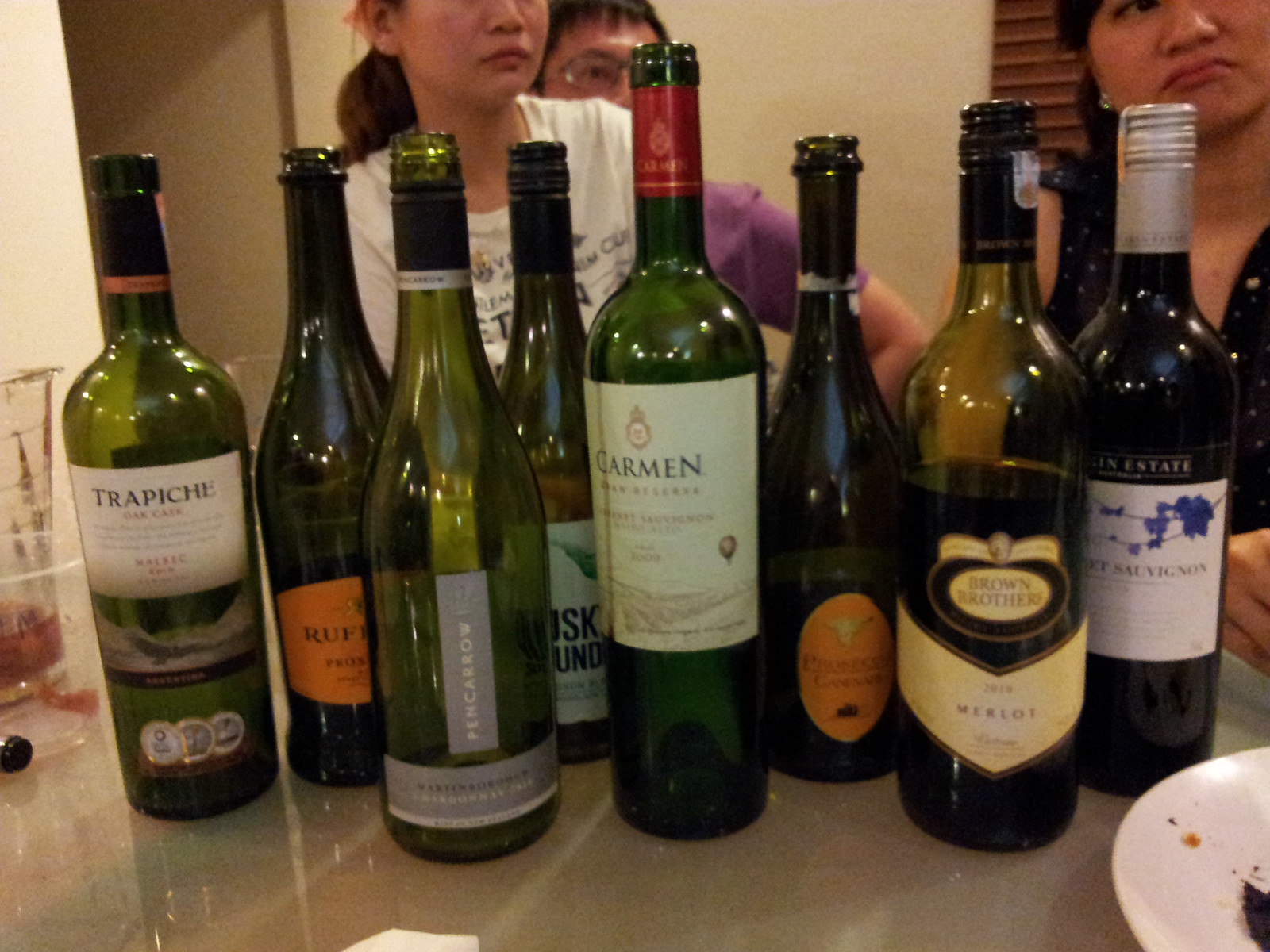The image is a low-resolution color photograph in landscape format, featuring eight wine bottles arranged in a line on a glass tabletop. The bottles, varying in color from greenish to yellowish tints, are mostly empty with their caps off, except for the two rightmost bottles. The labels identify some of the wines, including Trepacci, Ruffio, Pincero, Carmen, and Brown Brothers Merlot 2019. One of the unidentified bottles has an orange label, and another has a yellowish label. A white plate is visible at the bottom right, and a mostly empty plastic cup with a red drink is situated in the left-middle foreground. In the background, three people - likely women, possibly from an Asian descent and maybe Filipino - stand behind the bottles. One is a young girl in a white t-shirt with black writing, another wears a purple short-sleeved shirt, and the third person in the upper right corner sports a v-neck shirt, all of them looking towards the right side of the image.